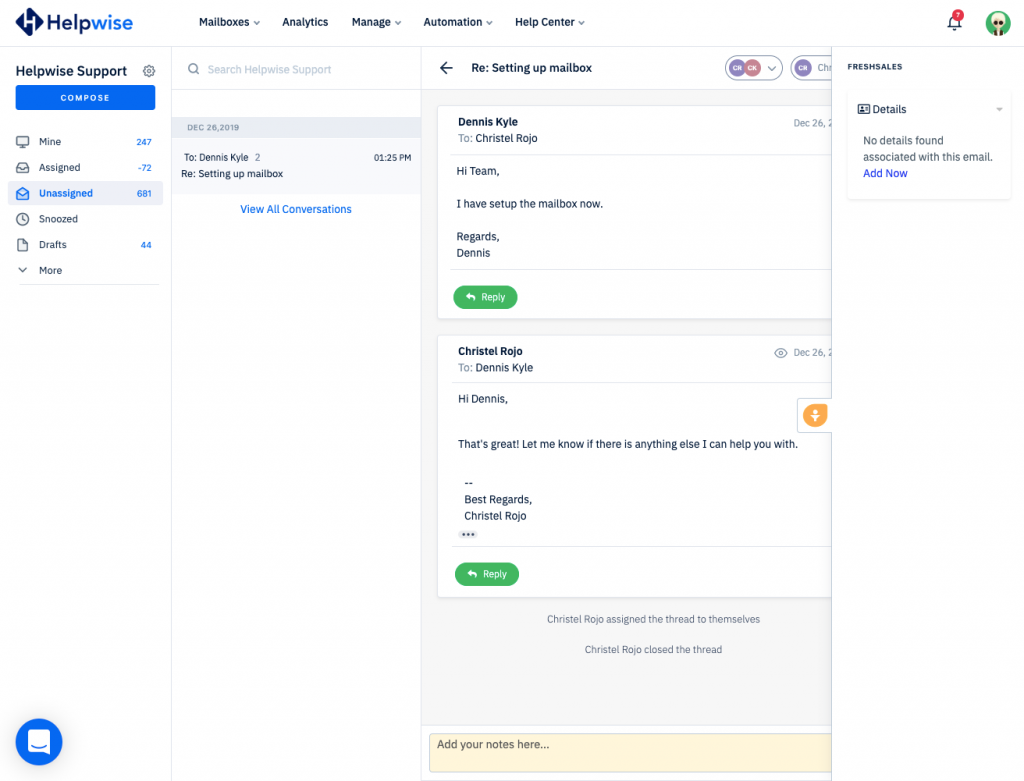The interface of a HelpWise account is displayed, structured in four distinct columns. In the top left corner, the HelpWise logo is prominently featured, with 'Help' in a dark navy blue and 'Wise' in a bright blue. Adjacent to the logo are five menu options: "Mailboxes" followed by a down arrow, "Analytics," "Manage" with a down arrow, "Automation" with a down arrow, and "Help Center" with a down arrow.

To the right of these options is a notification bell with a red dot, indicating an alert. Next to the bell is a white icon that alternates between an exclamation point and a question mark. Further right, there's a circular profile icon depicting a person wearing glasses and a black shirt.

The first column on the left lists the following items from top to bottom:
- "HelpWise Support" with a gear icon beside it.
- A blue rectangular "COMPOSE" button in white capital letters.
- A computer screen icon labeled "Mine" indicating 247 items in blue.
- An envelope icon labeled "Assigned" with a corresponding negative 72 in gray.
- An envelope icon highlighted in gray labeled "Open" with 681 unassigned items.
- A clock icon labeled "Snoozed."
- A page icon with a corner turned down labeled "Drafts," noting 44 drafts in blue.